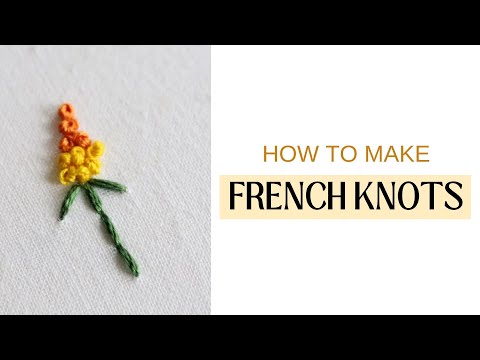The image shows the front cover of a book that provides instructions on creating thread-based artwork, specifically detailing how to make French knots. The cover has a simple design with two black lines, one at the top and one at the bottom. The space between these lines is divided into two sections: a grey portion on the left and a white portion on the right. The white section contains the text "How to make French knots," with "How to make" written in a light shade of orange (or gold) and "French knots" in larger black print. This text is also highlighted by a small pink box providing a pinkish backdrop. The grey section showcases an intricately detailed flower, with a green stalk and blossoms in shades of yellow and peach, all meticulously crafted to appear as if made from thread through techniques like knitting or crocheting, featuring French knots. The background fabric of the flower design is white, enhancing the contrast and intricacy of the artwork.